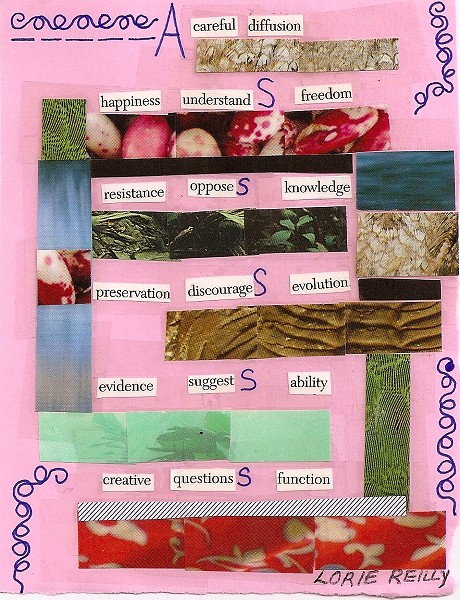This image features a handmade collage set against a vibrant pink construction paper background. The collage showcases an eclectic mix of objects and textures, arranged haphazardly without a centralized focus. Various materials are pasted onto the paper, including pieces of fabric, photos of everyday items like red-skinned potatoes, green leaves, a tan shell, and fields of green grass. Several patterns are hand-drawn with what appears to be a marker or crayon, adding to the artistic feel.

Scattered across the collage are small rectangular white boxes containing black text, snipped from other sources, and meticulously pasted on. These text snippets include words like "Careful diffusion," "Happiness," "Understand," "Freedom," "Resistance," "Oppose," "Knowledge," "Preservation," "Discourage," "Evolution," "Evidence," "Suggest," "Ability," "Creative," "Question," and "Function."

In the center of the image, there is blue handwritten text featuring the letters "A S S S S S," which adds a personal touch to the piece. The bottom right corner bears the creator's name, "Lori Riley," signifying authorship. Overall, the image conveys a whimsical and playful nature, reminiscent of a child's collage project, rich with colorful elements and insightful words interwoven throughout.